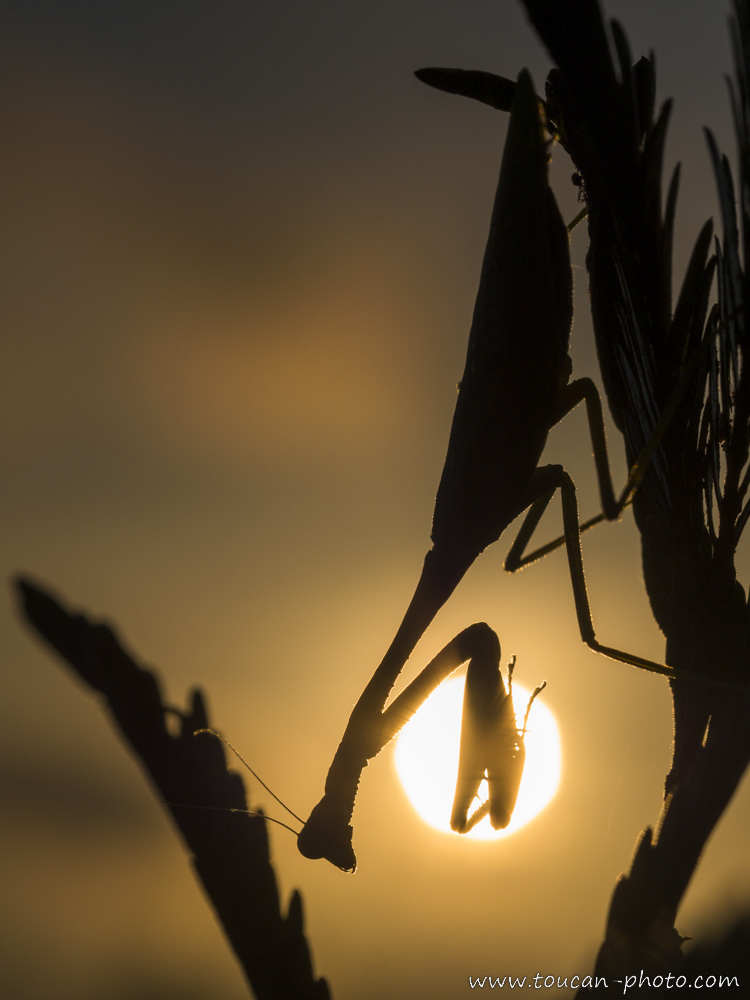This striking image captures a praying mantis hanging upside down on a plant, silhouetted against a dramatic sunset. The mantis is completely black, with its distinct body outline highlighted against the overcast, yellow-tinged sky. The sun, positioned near the horizon, casts a warm glow, transitioning from golden hues at the bottom to darker reds and browns towards the top. The focus of the photograph is sharp in the foreground, detailing the praying mantis's two antennae, nub neck, curved claws, and thin legs. The photograph's backdrop, however, is blurred, emphasizing the clarity of the silhouette. The image, which has the website www.toucan-photo.com inscribed in the bottom right corner, beautifully captures the serene yet evocative moment of nature at either sunrise or sunset.